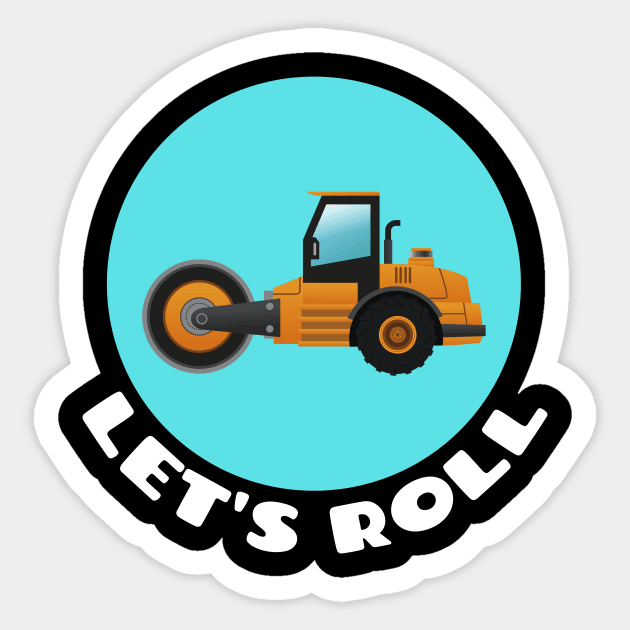The image features a circular sticker prominently displayed on a white square background. This sticker, intended as a logo, showcases a cartoon-style yellow steamroller, distinguished by its large black front roller and standard black rear wheel. The steamroller, complete with a driver’s carriage topped by a yellow roof and a black exhaust pipe curving to the right, faces towards the left. Surrounding the steamroller, the sticker has a light blue circular background. Encircling this scene, the sticker has a dual outline: an inner white border and an outer black border. At the bottom of the circle, the words "Let's roll" are boldly written in cartoonish white lettering, perfectly integrated into the design.